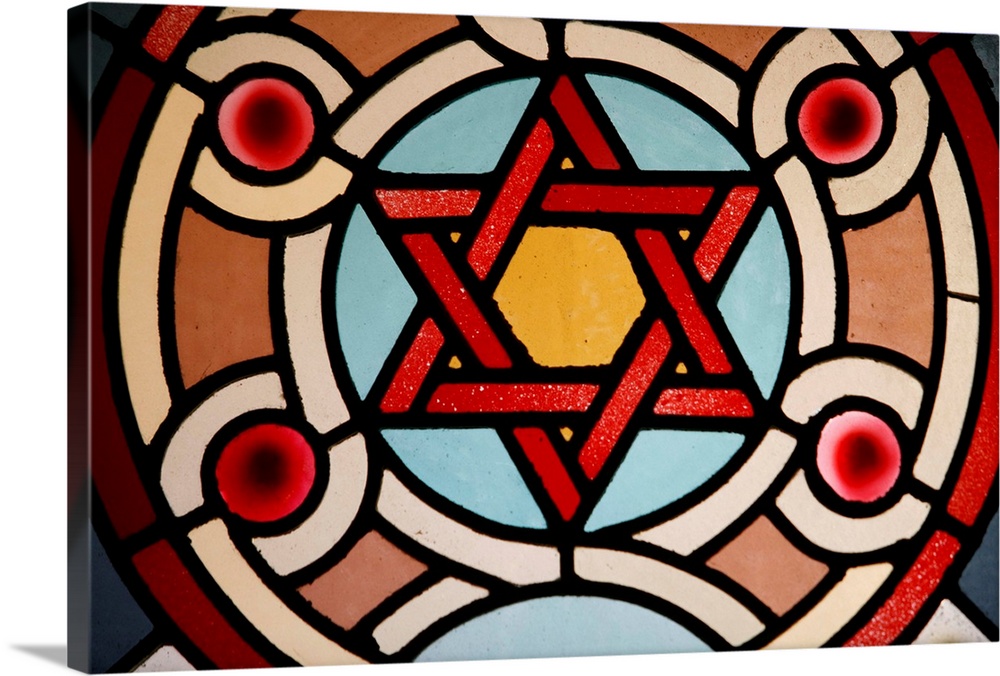This image resembles a stained glass artwork featuring a complex and detailed pattern centered around a Star of David. Starting from the outermost edge, the composition includes a circular border in varying shades of red. Just inside this red border is a whitish ring that transitions into the main pattern. 

The design primarily consists of concentric circular motifs and intricate segmentation. The outer circle is red with internal black segmentations, leading to a white ring with similar segmentation patterns. These segmentations create a repetitive, circular pattern that includes several smaller circles, yielding a sense of layered depth.

At the bottom of the larger pattern is a half-arch in light blue, bordered by white. Within this arch and extending towards the center are additional circular patterns, including another white ring that connects visually with the red-tinted smaller circles.

At the heart of the composition is the Star of David, formed by two overlapping triangles creating a pentagram. The pentagram's lines are segmented, and the intersections and gaps between the triangle lines are filled with yellow. Encircling the Star of David is a light blue ring, followed by an off-white beige ring, then a series of alternating dark and beige rings.

At four corners surrounding the Star of David, additional red circles sit in their own distinct rings, echoing the central design. The innermost part of the Star of David features a yellow hexagram, contrasting against darker maroon borders of the triangles.

The complex interplay of colors—reds, light blues, whites, beiges, and yellows—combined with the geometric segmentation and layering, gives the painting a vibrant, textural appearance reminiscent of stained glass.